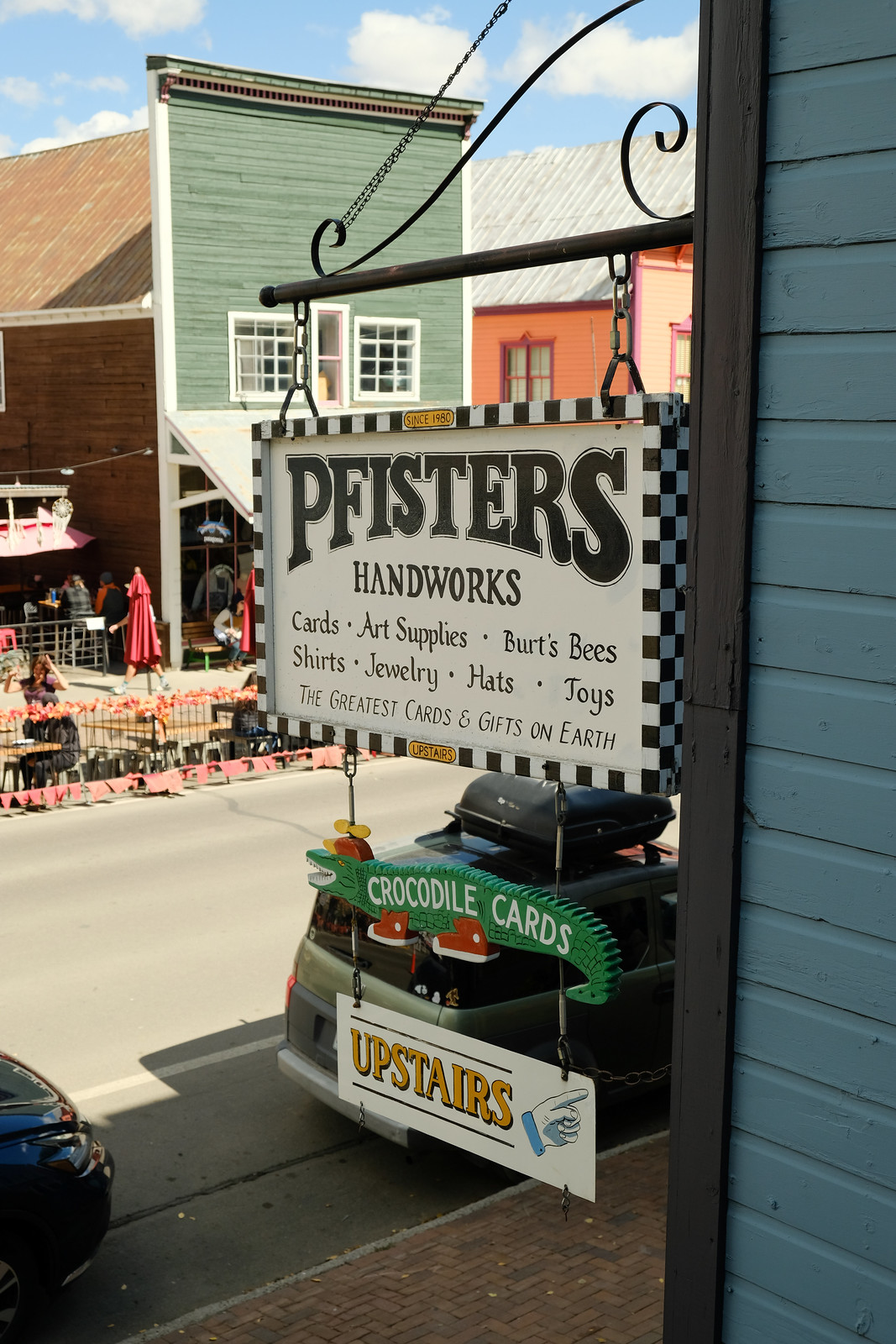The photograph captures a picturesque outdoor street scene in a small town, framed by a strikingly detailed handmade gift store sign. The perspective is as if from a doorway or corner of a blue-painted wooden building with black trim. The hanging sign, suspended by two chains from an iron wrought metal pole, showcases "P-F-I-S-T-E-R-S Handworks," offering items like cans, art supplies, Burt Bee shirts, jewelry, hats, toys, and much more. The sign, likely crafted from high-quality ceramic, is bordered by a distinct black and white checkered pattern. Beneath it, a green crocodile-shaped sign with a red hat reads "Crocodile Cards," and further down, another sign points upstairs with a beckoning hand.

The sidewalk below is constructed of brick and features a black and white checkered border. In the backdrop, a street runs by with parked cars lining its sides, and across the street, other wooden buildings, including a green one with white windows, add to the old-town charm. There is also an inviting patio area where people are leisurely seated, suggesting a café ambiance. The sky above is a bright blue adorned with patches of white clouds, further enhancing the inviting atmosphere of this quaint town scene.